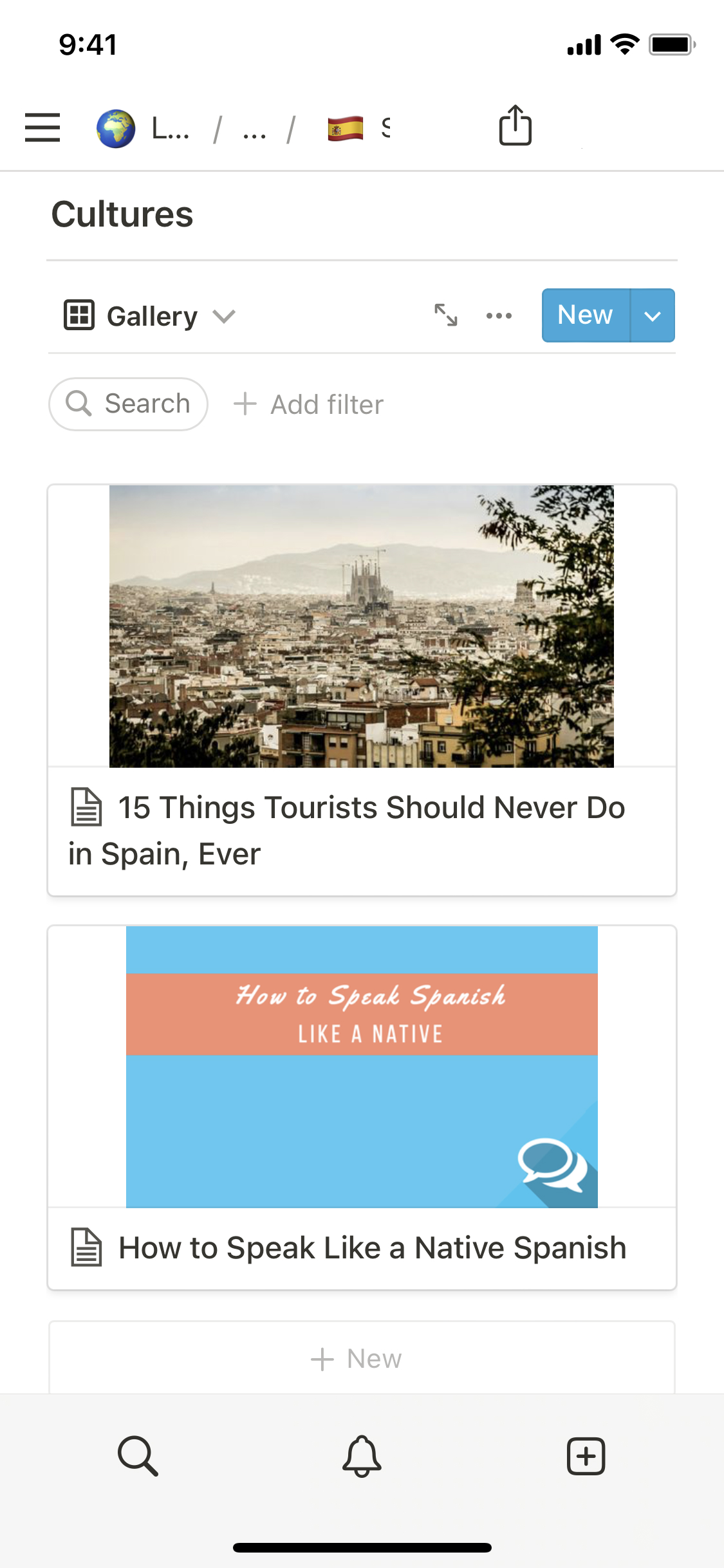The image is a screenshot from a mobile device with a clean white background. In the top-left corner, the screen displays the time "9:41" in bold black font. Moving to the right corner, there are icons indicating a full battery, strong Wi-Fi connection, and full internet signal. On the left side of the screen, three horizontal black lines are stacked, each about half an inch apart. Next to these lines is a globe icon, followed by a partially visible URL with ellipses and slashes ("L...\\/...\\/"), and a flag featuring a yellow center flanked by red at the top and bottom. Just below, the upper part of an "S" is visible before it vanishes into the background.

Further down, a download icon resides above a thin gray line. Bold black text on the left reads "Culture," followed by a thick gray line and the word "Gallery" alongside its respective icon. A dropdown tab with an arrow pointing diagonally up to the left and down to the right lies next to the icon. To the right of this, another set of three black dots and a blue tab labeled "New" appear, the latter with a white dropdown arrow.

Moving below, there is a search bar on the left with placeholder text "Search" and an icon, followed by the words "plus add filter." The main image shows an aerial view of a city, revealing rooftops, skyline, and trees along the sides. Beneath this cityscape image, bold black text reads "15 Things Tourists Should Never Do." Following this, in smaller font, it says "In Spain, Ever." Adjacent to the text, there is a PDF icon.

Below this section, a light blue square houses a smaller pinkish-tan rectangle. This rectangle displays the white text "How to Speak Spanish," followed by "Like a Native" beneath it. A bubble icon is situated in the bottom left corner of this area. In black text below, it repeats the phrase "How to Speak Like a Native Spanish." A small page icon appears to the left of this text, and the word "New" faintly in gray with a plus sign can just be discerned.

At the bottom, a notification icon is visible on the left, and a search icon at the left-middle area. On the right side, there is a white square with a gray border containing a gray plus sign. The bottom part of the image features a thick dark blade-like or black-tie-shaped border stretching horizontally.